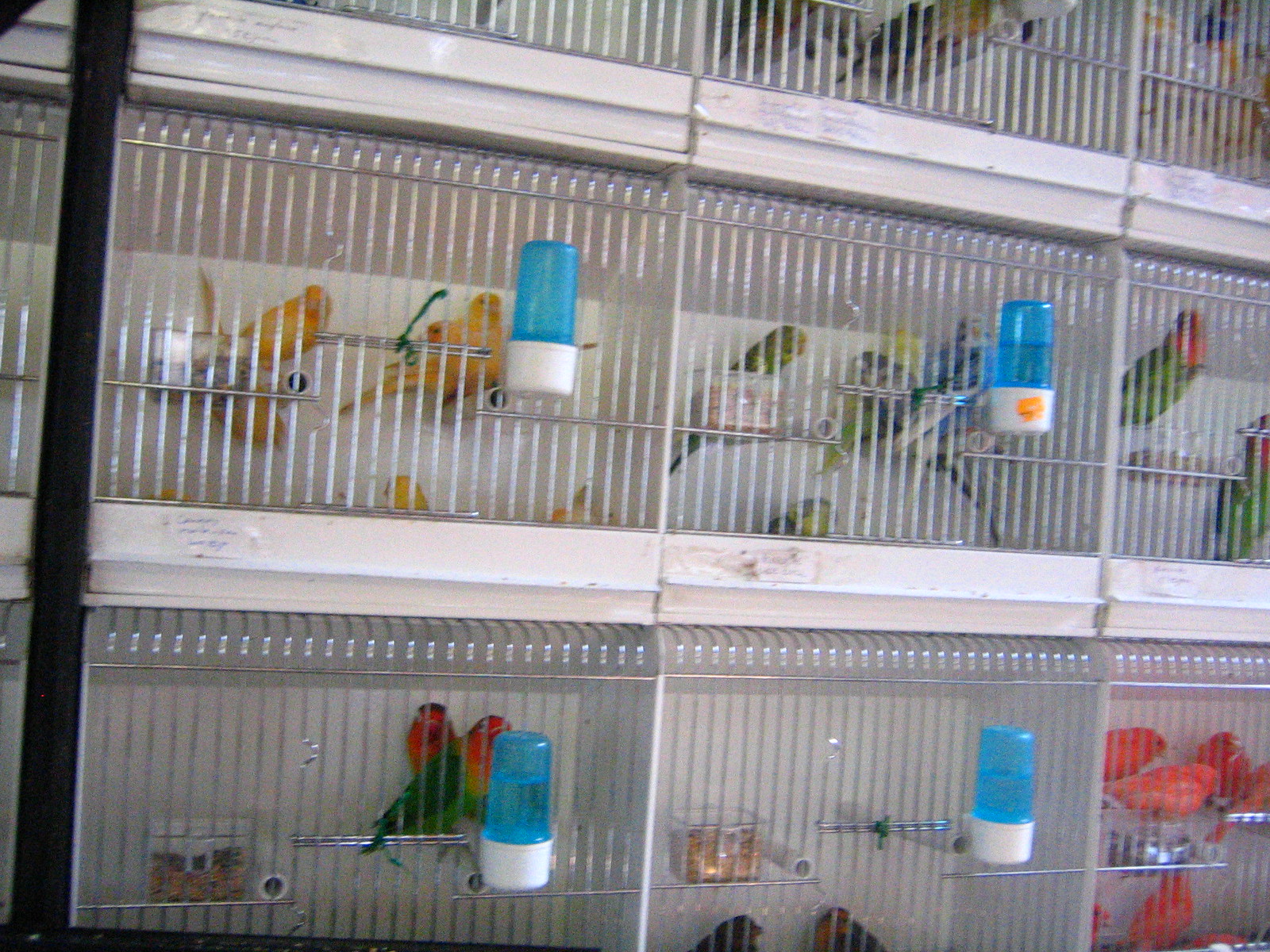The image depicts a wall inside a pet shop, where numerous bird cages are stacked one atop another, extending both upwards and to the left and right, with the topmost row partially out of frame. The cages, made of white or silver wire, house an array of small finch-type birds of various vibrant colors. These include entirely red birds, green-bodied birds with red heads, yellow birds with hints of orange, and multicolored birds with combinations of red and green. Blue plastic water bottles are affixed to the front of each cage, providing drinking water for the birds. Some cages have labels on them, likely indicating the species or breed of the birds contained within.